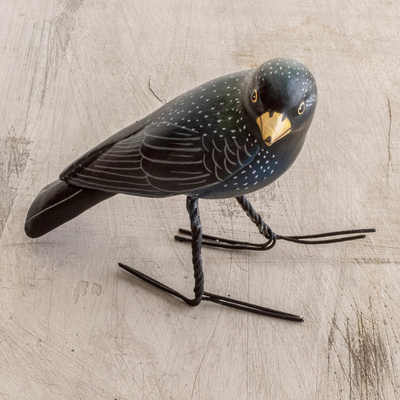This image captures a detailed, overhead view of a craft-like bird statue with an intricate design. The bird’s body is predominantly dark blue with stylized white specks adorning its head, back, and chest. It features a vibrant yellow beak and sharp yellow eyes. The legs and feet appear crafted from twisted black metal or wire, with the feet positioned straight ahead and behind, enabling the bird to stand independently. The statue rests atop a light-colored wooden surface, possibly a table, which has a somewhat scratched and worn appearance. The distinct interplay of colors and materials gives the bird a striking, almost lifelike presence while maintaining an artistic, handmade charm.